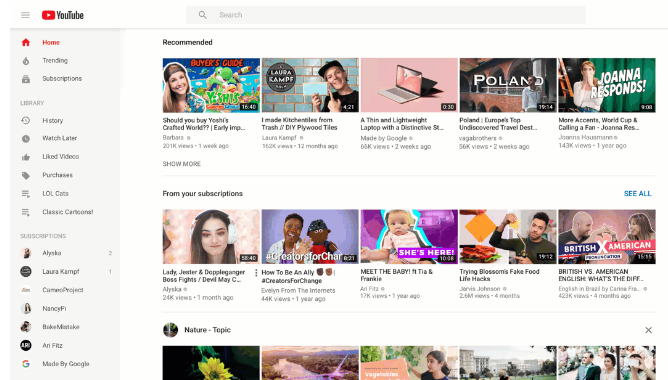The image depicts a YouTube homepage with the menu bar extended from the top left corner. At the upper-left side, there is the iconic red rectangle with a white play button, which is the YouTube logo, followed by the word "YouTube" in black text. The extended menu showcases various options: Home, Trending, Subscriptions, Library, History, Watch Later, Liked Videos, Purchases, LOL Cats, Classic [something], and Cars [something]. The highlighted option in red is "Home," indicating the user is currently on the home page.

The main section of the page is divided into noteworthy segments. Under "Recommendations," there are five video thumbnails displayed in a row. The titles of these recommended videos are:
1. "Should you buy Yoshi's Crafted World: Buyer's Guide"
2. "I Made Kitchen Lists from Trash: DIY Plywood Tiles"
3. "A Thin and Lightweight Laptop with Distinctive [something]"
4. "Poland: Europe's Top Undiscovered Travel Destination"
5. "More Accents: World Cup and Calling a Fan"

Below the "Recommendations" section is another segment titled "From Your Subscriptions," showing another set of five videos in a row. Further down, under the section named "Nature Topic," five more videos are presented in a row. The detailed layout and highlighted content provide the user with a clear and organized browsing experience on the YouTube homepage.